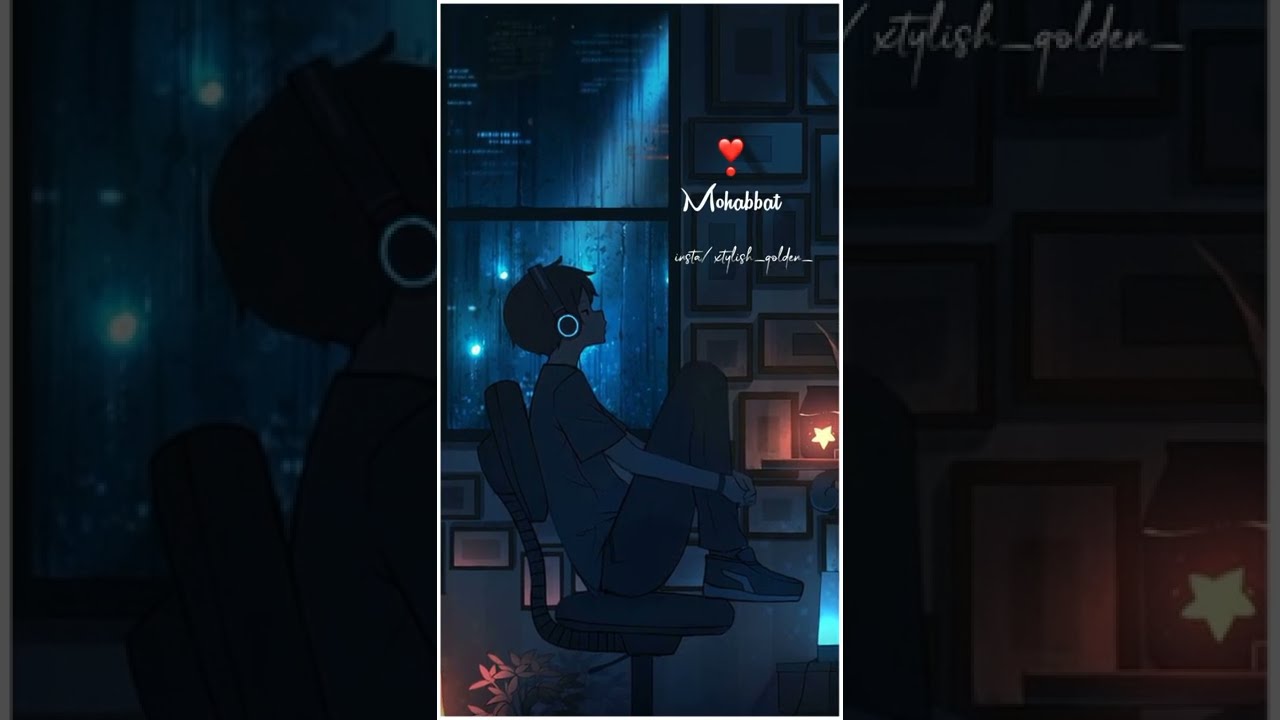The image depicts a teenage boy with short dark hair, sitting cozily in a black office chair at a slight angle, likely engaged with a computer or desk in front of him, though the object is cut off from view. He is wearing a t-shirt, jeans, and tennis shoes, with over-the-ear headphones that have a bluish circular detail at the speakers. His body posture is quite relaxed, with his feet perched on the edge of the chair and his arms wrapped around his legs, bringing his knees close to his chin. The room he occupies appears dimly lit, enhanced by the soft glow of light streaming through a window to the front, emphasizing the rainy scene outside with water trickling down the glass. The background reveals a glimpse of city skyscrapers, suggesting a large urban setting. Surrounding him are various details, including a plant near the floor, multiple pictures adorning the wall, and text in the top right corner reading "Moe Hobbit" or "Mokabot." The image captures an artistic and somewhat melancholic mood, fitting for an album cover or a stylized social media post, marked by a distinctive red heart with a corresponding red dot below it.